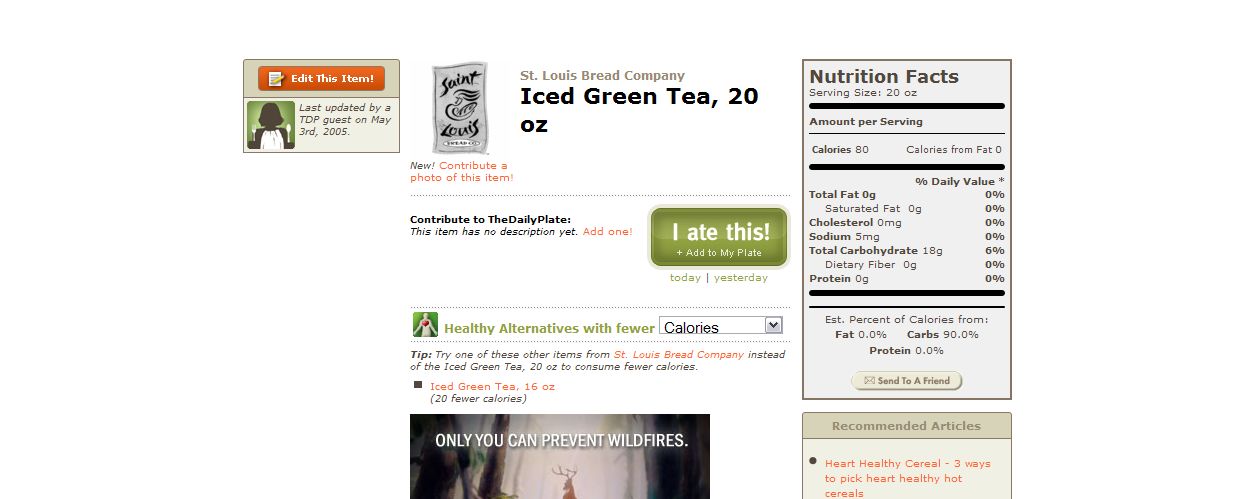The image appears to showcase a menu or nutritional information for a beverage at the St. Louis Bread Company. In the top left corner, there is an orange rectangle with the text “Edit this item,” noting that a TDP guest updated the listing on May 2nd, 2005. Centered at the top of the image, the name "St. Louis Bread Company" is displayed in black text, above an item labeled "Iced Green Tea, 20 ounces."

On the right side of the image, black text encourages users to "Contribute to the Daily Plate," alongside a green rectangle that reads "I Ate This" in its center. In the bottom left corner, there's a section labeled "Healthy Alternative with Fewer Calories," offering a tip to try one of the items listed below: "Iced Green Tea, 16 ounces, 24 calories." Beneath this is an advertisement with a message, "Only You Can Prevent Wildfires," featuring an image of a deer.

To the right, nutrition facts for the 20-ounce serving of Iced Green Tea are provided. The details include:
- Calories: 80
- Calories from fat: 0
- Total fat: 0 grams
- Saturated fat: 0 grams
- Cholesterol: 0 milligrams
- Sodium: 5 milligrams
- Total carbohydrate: 16 grams
- Dietary fiber: 0 grams
- Protein: 0 grams

At the bottom of the image, there are references to bread commercials, heart-healthy cereal, and various ways to select heart-healthy hot cereal.